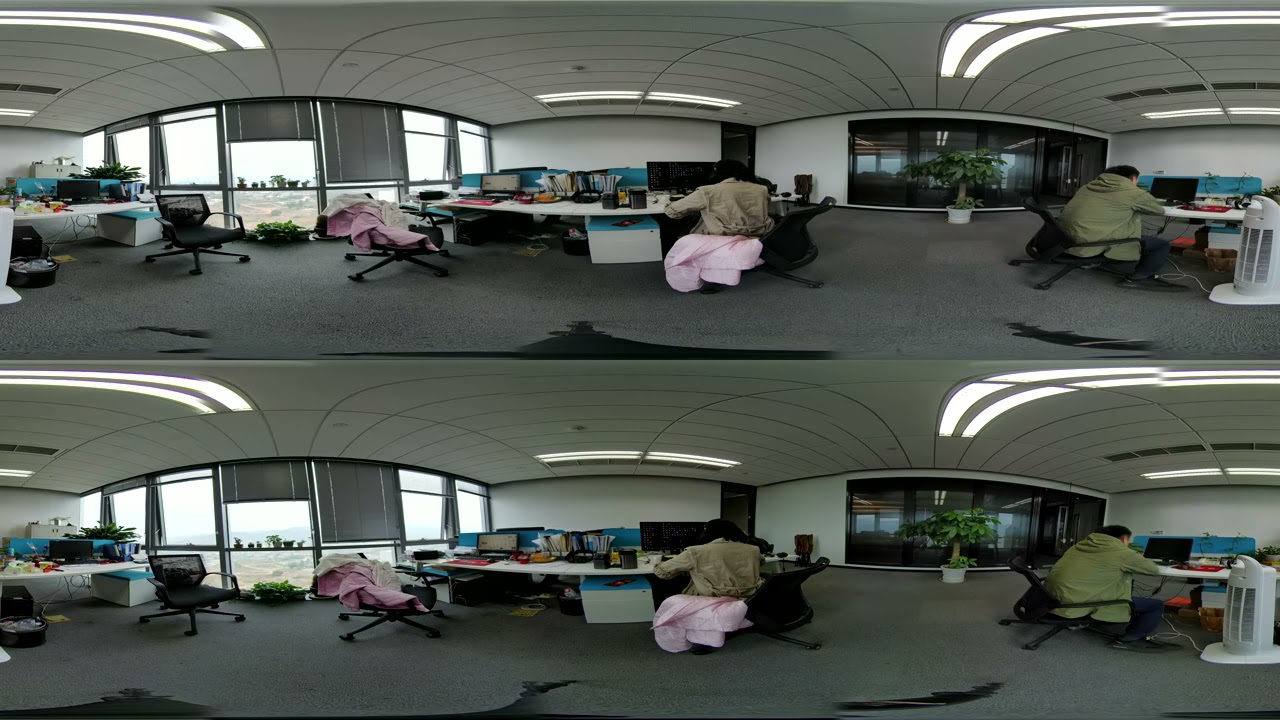This peculiar image features two nearly identical photographs layered on top of each other, creating a distorted, wide-angle view. It captures a casual office environment, seemingly with a lenient dress code. In the foreground, on the left side, a man in a pale green jacket, appears in both layers of the image, though the lower one is slightly brighter. Adjacent to him on the right is a device resembling an air purifier. Further back, there's a glass-walled room, partially obscured by a potted plant that is positioned to the side of what appears to be a tree. On the right side of the image, another person is seated at a desk, dressed casually in a pale brown jacket and seated in a computer chair with a pink cover. The office features carpeting, ceiling lights that appear curved due to the distortion, windows to the left side covered with drapes allowing sunlight to filter in, blocked windows to the right, creating an interplay of natural and artificial lighting. The scene is set indoors, likely in the middle of the day, characterized by a palette of colors including gray, white, blue, orange, yellow, black, pink, and light blue. No text is present in the image, which interestingly contains no descriptive text, just an elaborate visual of a typical albeit unorthodox modern office setting.